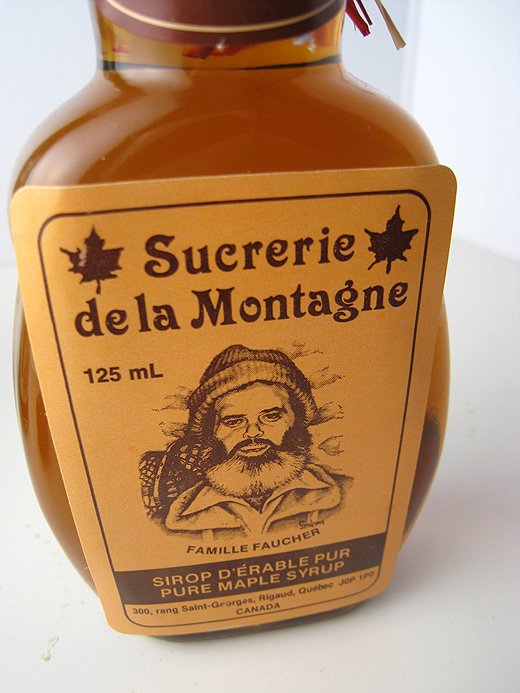The image features a brown glass bottle with a light brown label, prominently displaying a product name, "Sucrerie de la Montagne." The label, intricately detailed, includes an illustration of a man with a thick gray and black beard, wearing a beanie and a heavy coat. The man is smiling warmly at the viewer. Below his illustration is a black rectangle with the text "Pure Maple Syrup." The maple syrup, evidently labeled as Canadian with the iconic maple leaf, sits on a white surface, emphasizing its cultural authenticity.